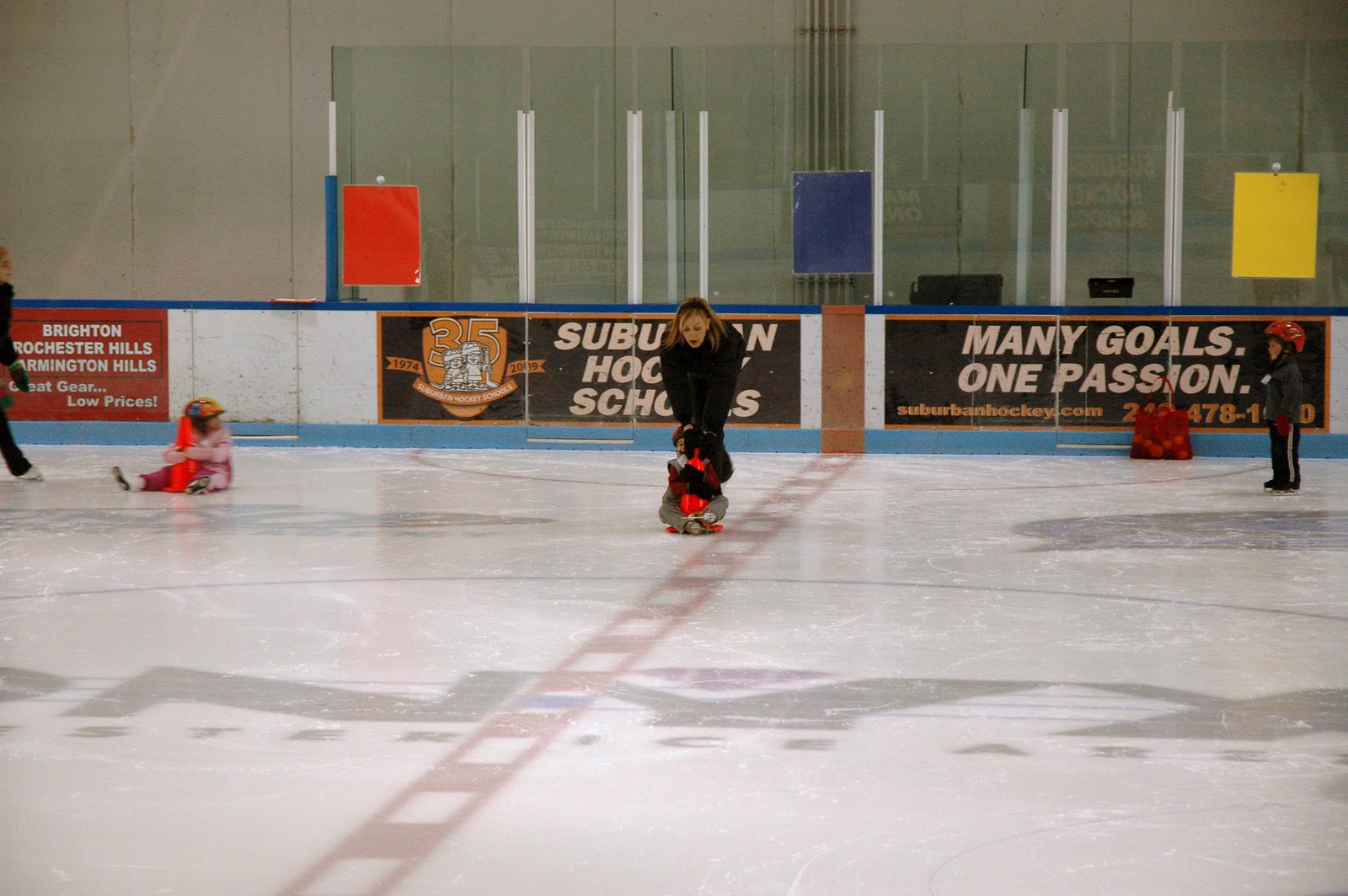In this photograph of an indoor ice rink, we see a dynamic scene featuring five individuals amidst a playful moment. At the center of the image stands a blonde woman in a black jacket, facing the camera. She is pushing a young child wrapped around a bright orange traffic cone across the ice. The child, equipped with a helmet, seems to enjoy the ride as they glide over the red line marking the rink's halfway point.

To the right of the central pair, another boy with a helmet and ice skates stands independently on the ice. On the left, a little girl in a pink outfit and a rainbow-patterned bike helmet sits on the ice, clinging tightly to a white traffic cone. Further left, partially out of frame, is another adult in black, suggesting another supervisory presence.

The rink's background features a glass panel adorned with several vertical white stripes and three colored rectangles—red, blue, and yellow—adding a colorful backdrop to the scene. Beyond the glass, a white wall with multiple doors completes the setting, highlighting the structured environment of the ice rink. This image captures a moment of joy and learning, as both adults and children engage in a shared activity on the ice.